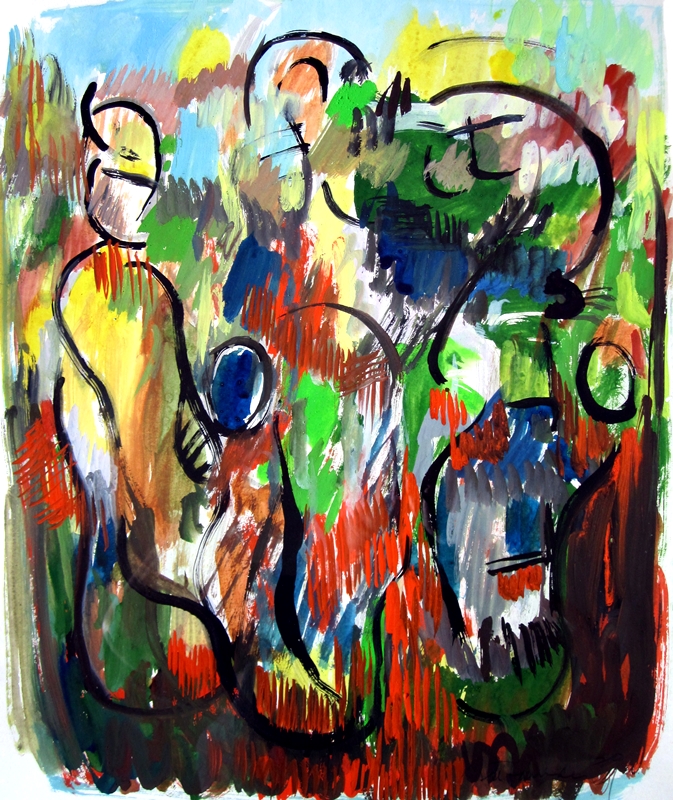This contemporary and vividly colorful abstract painting is slightly taller than it is wide. The artwork features a vibrant array of hues including blue, yellow, pink, red, green, lime green, dark brown, and dark blue, applied in thick, vertical brushstrokes and slashes that create a dynamic, chaotic background. The foreground is adorned with loosely drawn, rounded-edged silhouettes of what appear to be three human figures, outlined in black ink or paint. These simple, almost scribble-like figures stand in a row, their heads and bodies discernible but lacking detailed features or limbs. The overall composition, a blend of bold colors and abstract forms, evokes a lively, enigmatic scene that leaves much to the viewer's imagination.